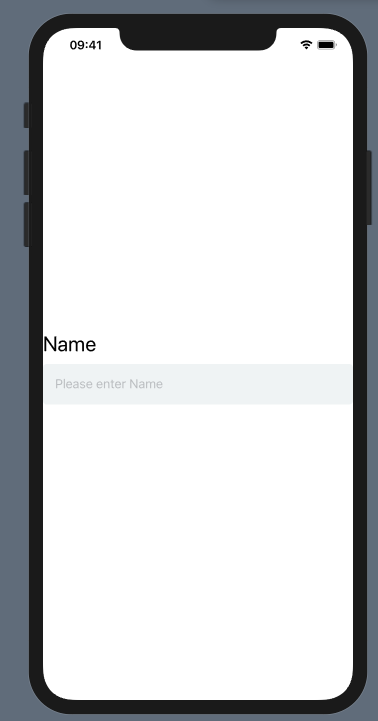The image features a smartphone set against a gray background, highlighting the silhouette of the device. The phone has a prominent black border, suggesting it is encased. On the left side, three buttons are visible, while a single button can be seen on the right side. The screen of the phone is primarily white, with minimal text displayed. At the top of the screen, "9:41" is displayed in black numbers, with no indication of AM or PM. To the right of the time, the phone shows full signal strength bars and a fully-charged battery icon, though the phone is not plugged in, as indicated by the absence of a charging symbol.

The interface on the screen is simple: the top and bottom parts of the display are white, with a gray input field situated in the middle. Above this field, the word "Name" is prominently displayed in larger letters. The gray field below it contains the placeholder text "Please enter name," which stands out against the otherwise white screen. The black border of the phone case slightly covers the top part of the screen, encroaching between the time display and the signal and battery indicators.